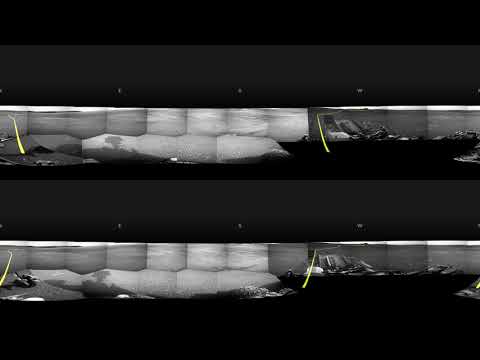The image consists of three horizontally aligned panels with predominant black and white tones. The top third of the image is predominantly black, while the bottom two panels, one slightly above the other, contain various shades of gray. Upon closer inspection, these lower panels feature subtle differences but largely share similar visual elements. Each of the two bottom panels displays what appears to be a horizontal figure, potentially a boat, on the right side, towing an indistinct object on the left. Both panels are cut off by a black band at the bottom.

Intertwined with these panels are visual elements resembling gray bars segmented by puffier, lighter shapes. These bars show a gradient from regular gray on the left, very light gray in the middle, to dark gray on the right. Scattered atop these bars are three light gray dots, possibly rivets or stars, though this remains uncertain. Additional details such as yellow poles and lime green streaks further complicate the visual narrative but are not easily discernible due to the overall blurred and dark quality of the image. In some sections, the figures bear resemblance to an abstract or blown-up area, possibly akin to the exterior of a bouncy house, incorporating pointy angles and white and gray worm-like shapes. The overall ambiguity of the image, combined with the mix of black bands and visually indeterminate motifs, leaves much open to interpretation.